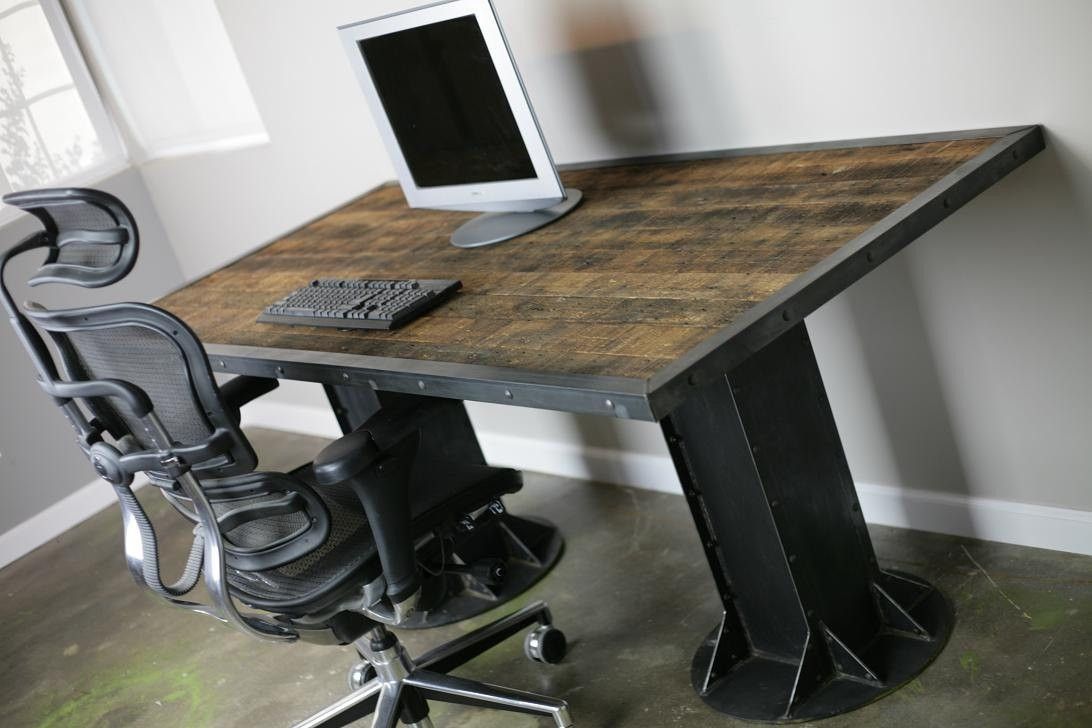The photograph captures a home office environment featuring a substantial wooden-top desk supported by bulky, I-beam-like legs, giving it a robust and immovable appearance. Atop the desk, there is an old-fashioned, square, flat-screen monitor and a wireless desktop keyboard. In front of the desk stands a modern, high-tech office chair with a mesh design and a high backrest equipped with a neck cushion. The image is slightly tilted about 20 degrees to the right, providing an unconventional perspective. The backdrop includes windows that allow a good amount of natural light to illuminate the space, casting a mixture of gray, black, silver, white, brown, and pewter hues across the scene. The floor appears to be a plain, non-carpeted surface. The overall composition of the photo excludes any text and focuses purely on the elements within the room.